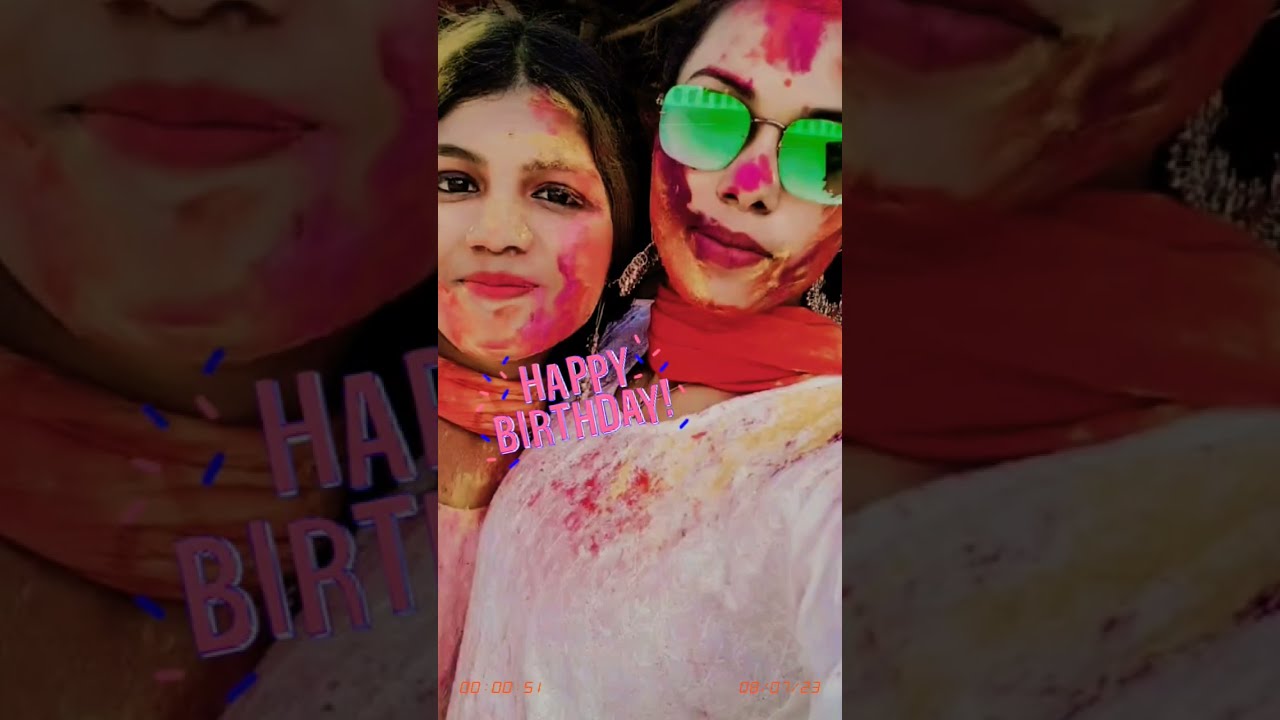In this vibrant, close-up photograph, two young women, likely around 18 or 19 years old, are captured joyously celebrating a special birthday occasion. Both are adorned with vivid red scarves around their necks and are playfully smeared with colorful powders, hinting at a fun-filled event like a color run or a festive powder blast. The woman on the right, wearing large circular sunglasses with reflective green lenses, is dressed in a white blouse speckled with paint. The woman on the left, with long dark brown hair parted in the middle, sports a pink shirt. Their faces are splashed with shades of pink and orange, while yellow, red, and pink powders cover their tops. Superimposed between their closely pressed faces is a cheerful "Happy Birthday" caption in pink text, encircled by blue and pink confetti. The image, with its overexposed, enhanced colors, creates a lively, celebratory atmosphere. The edges feature parts of the central image, enlarged and faded to form a creative border. Additional details like timestamps "0000 051" on the lower left and "080723" on the lower right suggest this is a screen capture, likely from a TikTok video commemorating this joyful moment.